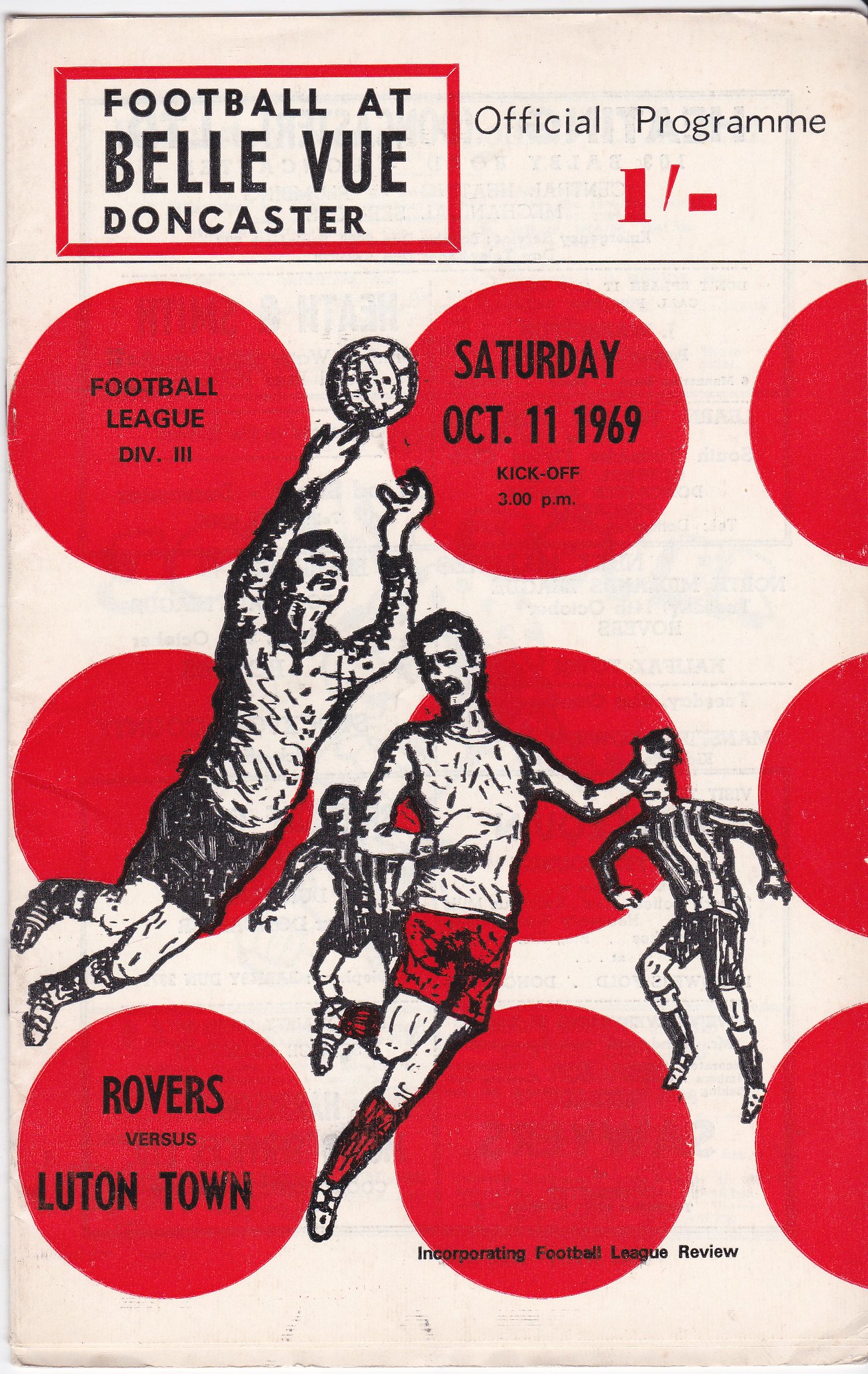The program for a soccer event features a light cream-colored background. At the top left corner, there is a red outlined box with black text that reads "Football at Bellevue Doncaster." Adjacent to this, on the right side, "Official Program" is printed in black text. Below these headings, there is a white number one within a small red rectangle, followed by a quote mark. Surrounding this are several red circles with details: the upper left circle says "Football League Division Three," the next circle states "Saturday, October 11, 1969. Kickoff 3 p.m.," and the bottom left one reads "Rovers vs. Luton Town." The bottom right circle contains the text "Incorporating Football League Review."

Centrally featured are black illustrations of animated characters engaged in a soccer game. The leftmost figure appears to be leaping through the air with arms extended upwards towards a soccer ball. Positioned behind him is a player in a jersey with black stripes, who seems hunched with arms slightly outstretched. To the right is another player bending his body towards the right while facing left, wearing red shorts and socks, with elbows bent and arms directed right. On the far right, partially obscured, is a player in a black and white striped jersey, whose head is blocked by the hand of the central player.